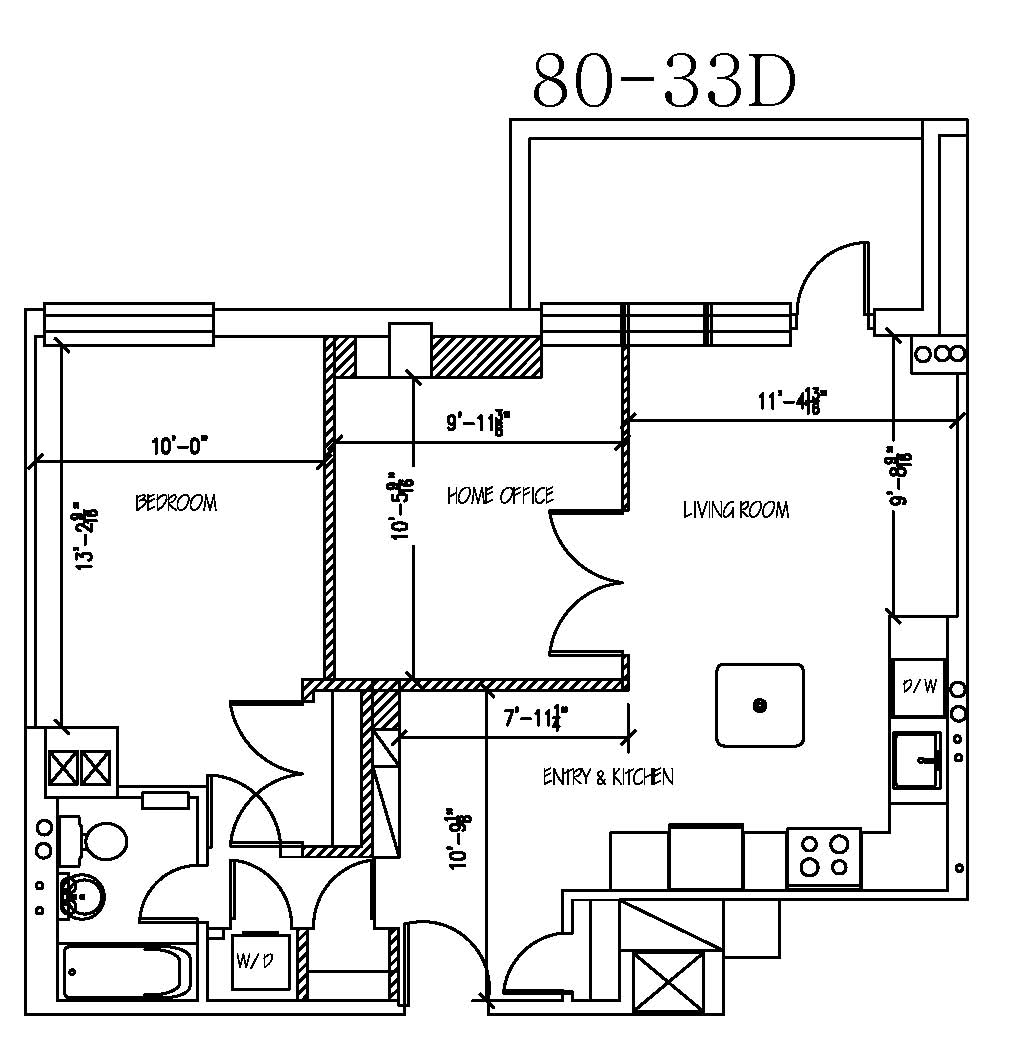This detailed floor plan, labeled with the designation "80-33D," showcases a thoughtfully designed home layout. At the top of the plan, we find a cozy porch area, leading through a door into a spacious living room. This living room features an open floor plan that flows seamlessly into the kitchen area, which is well-appointed with a center table, dishwasher, sink, stove, and refrigerator. The kitchen layout incorporates a slight left turn, where another door provides access to the outdoor space.

Adjacent to the living room are two large, swinging doors that open into a 9 feet by 11 feet home office, providing a dedicated workspace. Moving from the open kitchen and living area toward the left, a hallway leads to the bedroom. Directly ahead in the hallway lies a well-equipped bathroom featuring a toilet, sink, and tub. Additionally, there's a designated area for a washer and dryer, adding convenience.

The bedroom itself, positioned across from the home office but not connected by a door, offers ample space and includes a generously sized closet. This floor plan ensures a functional and comfortable living experience, with every detail meticulously considered.